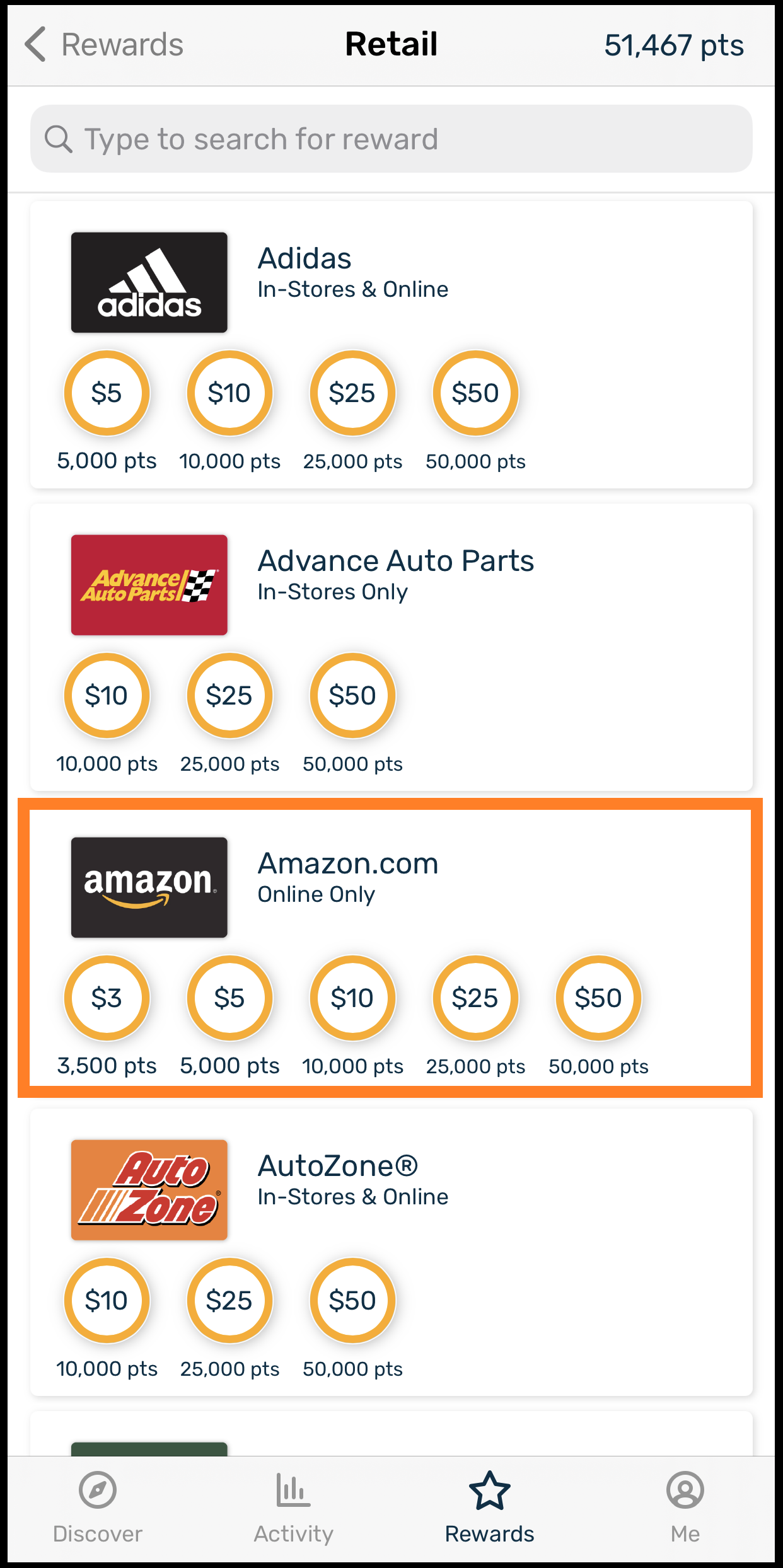This screenshot captures the "Reward Points" page from a retail platform. At the top center, a gray bar with the label "Retail" stretches across the screen. On the right side of this bar, a numerical display shows "51,467 points." To the left, the bar contains a "Rewards" label alongside a back button. 

Beneath this, there is a gray search bar prompting users to "Type to search for a reward." Following the search bar is a list of various gift cards, each accompanied by a monetary value inside an orange circle, and below each value, the corresponding cost in points. 

The available gift cards are from brands such as Adidas, Advance Auto Parts, Amazon, and AutoZone. For Adidas, the monetary values and corresponding costs in points are displayed as follows: $5 for 5,000 points, $10 for 10,000 points, $25 for 25,000 points, and $50 for 50,000 points. 

Towards the bottom of the screen, another gray bar features options labeled "Discover, Activity, Rewards, and Me," each represented by an icon.